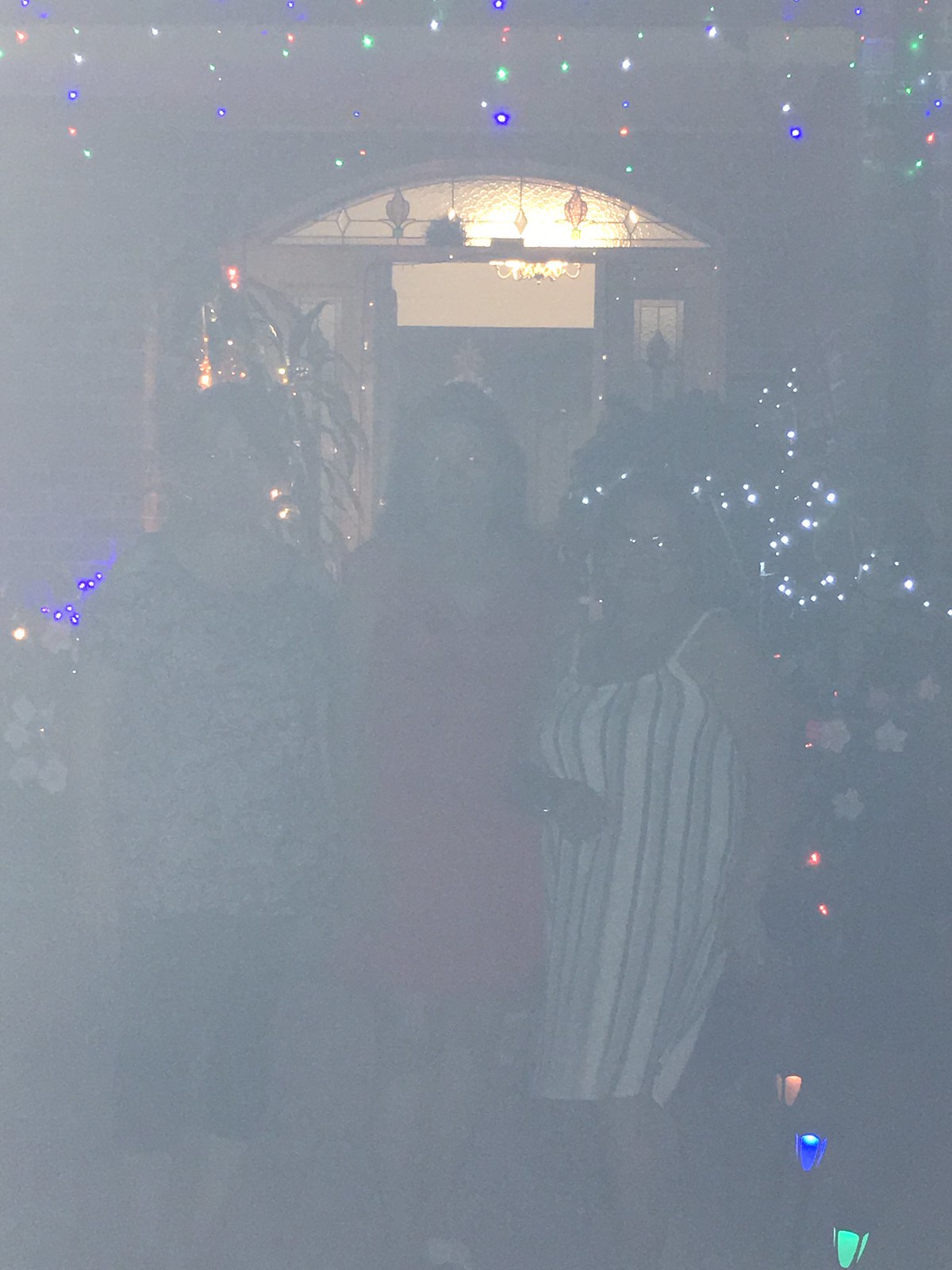In this slightly dark and somewhat low-resolution image, three women are posing closely together in front of a home's entranceway. The woman on the right is dressed in a white dress adorned with gray stripes and she is also wearing glasses. The woman in the middle stands out in a vibrant red dress. To the left, the third woman is dressed in a short-sleeved top paired with black pants and has short hair parted down the middle. She is also wearing glasses. Additional details in the background include a bush with flowers visible on the right side, adding a touch of nature to the scene.